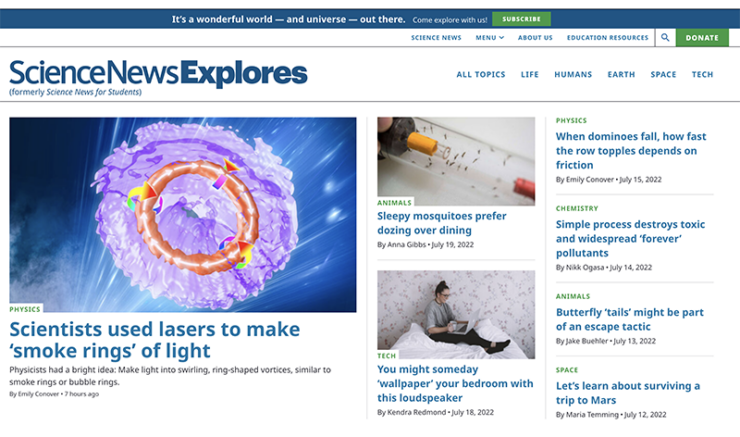This is a screenshot of a website with a clean, white background. At the top of the page is a dark blue navigation bar with white text that reads "It's a Wonderful World - and Universe - Out There. Come Explore with Us!" To the right of this text is a green button with white font labeled "Subscribe."

Below the navigation bar, the white background continues, featuring three dropdown menus labeled "Science News," "Menu," and "About Us," all in blue font. Next to these menus is a link labeled "Education Resources," followed by a blue magnifying glass icon representing the search function. Further to the right is another green button with white font that says "Donate."

Under these elements is the name of the website: "Science News Explorers, formerly Science News for Students." Adjacent to the site name is a menu listing the categories "All Topics," "Life," "Humans," "Earth," "Space," and "Tech."

In the lower-left corner of the screenshot, there is an article preview, which includes a photo featuring a green circle surrounded by blue bubbles. The headline of the article reads, "Scientists Use Lasers to Make Smoke Rings of Light."